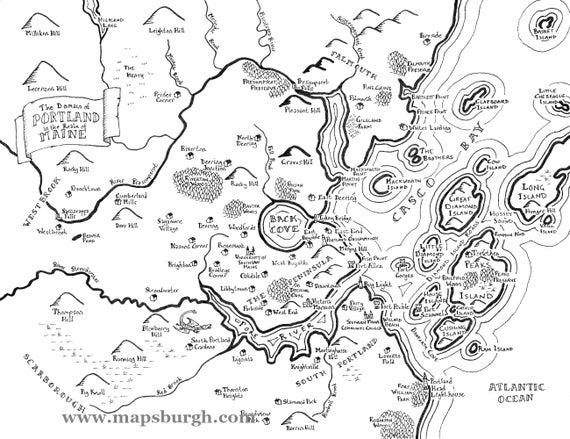This horizontal rectangular image is a detailed black and white map of the Portland, Maine area. It prominently features a curved banner in the upper left corner that reads "Portland, Maine." The map includes various topographical elements such as mountains and rivers, accurately depicting the region’s diverse landscape. Casco Bay, along with its numerous named islands including Long Island and Little Diamond Head, is prominently displayed, indicating the coastal nature of Portland. Bodies of water like Black Cove and Fore River are clearly marked, along with other geographical features such as inlets and coves. Small icons indicate towns, houses, and further natural features. The Atlantic Ocean is labeled in the bottom right corner. Finally, the map credits www.mapsburg.com as its creator, with this web address appearing as a watermark in the bottom left corner.